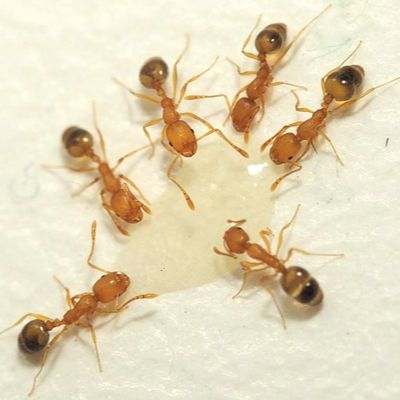The image depicts six orangish-brown ants with black-tipped abdomens, gathered together on a white, grainy crystalline surface that resembles salt or sugar. Arranged in a semi-circle, the ants have their heads pointed inward toward what appears to be a small recessed area in the center, possibly containing a sugary solution they are feeding on. Each ant displays distinct segmentation, black eyes, and slender, tapering limbs. The detailed arrangement of the ants shows two facing the lower right, one towards the lower left, while four others have their abdomens pointing towards the upper-left and upper-right corners. The scene evokes the sense of active, purposeful movement as the ants appear to be collecting the substance to take back to their nest.